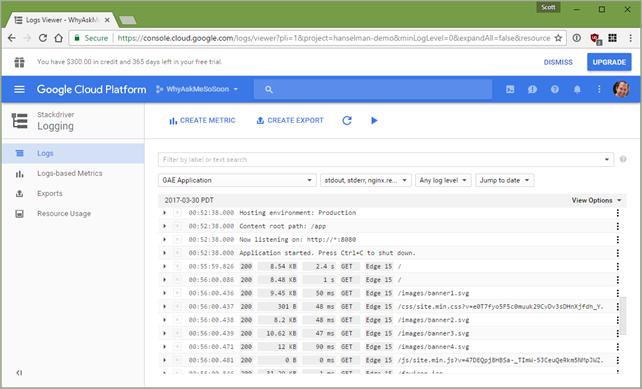The image displays a screenshot of a browser window with the Logs Viewer tab open. At the top of the browser, the tab title clearly reads "Logs Viewer," and the web address shown is console.cloud.google.com. Just below the browser address bar, a notification informs the user that they have $300 in credit and 365 days remaining on their free trial.

The interface prominently features the Google Cloud Platform logo on the left-hand side, horizontally aligned with a user profile picture on the right side. Directly beneath the Google Cloud Platform bar runs a vertical navigation menu on the left. This menu includes several options such as "Logs" with a subcategory "Logs-based metrics," "Exports," and the final option "Resource usage."

On the right side of the screen, the central portion is dedicated to logs information, displaying detailed log entries and associated data, which is the primary focus of the Logs Viewer tab.